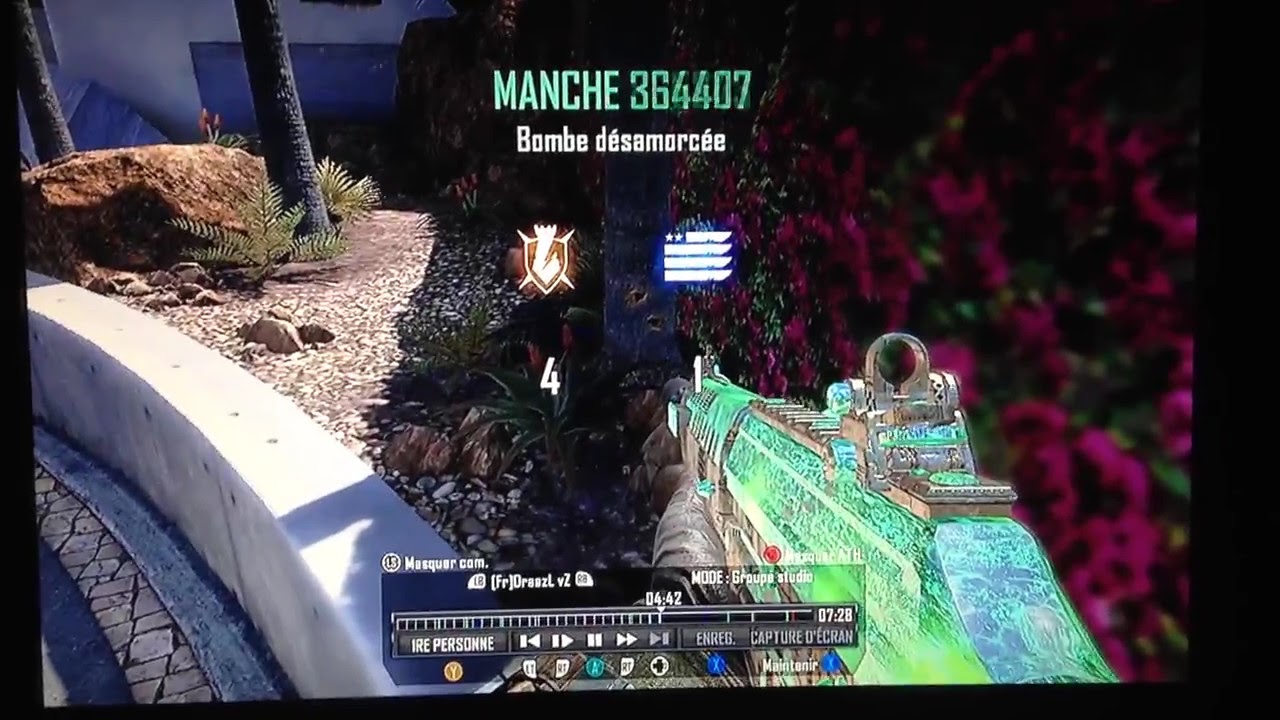In the detailed screenshot from a first-person shooter video game, the scene vividly showcases the player's perspective as they navigate the virtual environment. The primary focus is a vibrantly colored machine gun, predominantly bright green with hints of blue and yellow, suggesting a radioactive or nuclear aesthetic. The player, whose right hand is clad in a black glove, holds the weapon, aiming it toward a distant black rock.

To the left of the screen, there’s a curving slab of a concrete wall, signifying some form of cover or corner. Beyond the black rock, the landscape features a mix of brown soil, green plants, and a couple of trees with a brown rock nestled between their trunks. There are purple flowers visible to the right of the gun, adding a touch of color to the rugged terrain.

The top of the screen displays the text "Manche 364-407 Bombay de Saint Marseille" in lime green, suggesting the game is possibly set in a French context. Beneath this, a brown shield icon displays the number four, flanked by a flag marked with four white lines and two white stars. At the bottom of the screen, a gauge resembling a DVR playback bar indicates the mode of the game, accompanied by some unreadable statistical data, likely pertaining to the player's performance.

The entire image is bordered by black rectangles on all sides, further intensifying the immersive experience of this computer-generated environment.